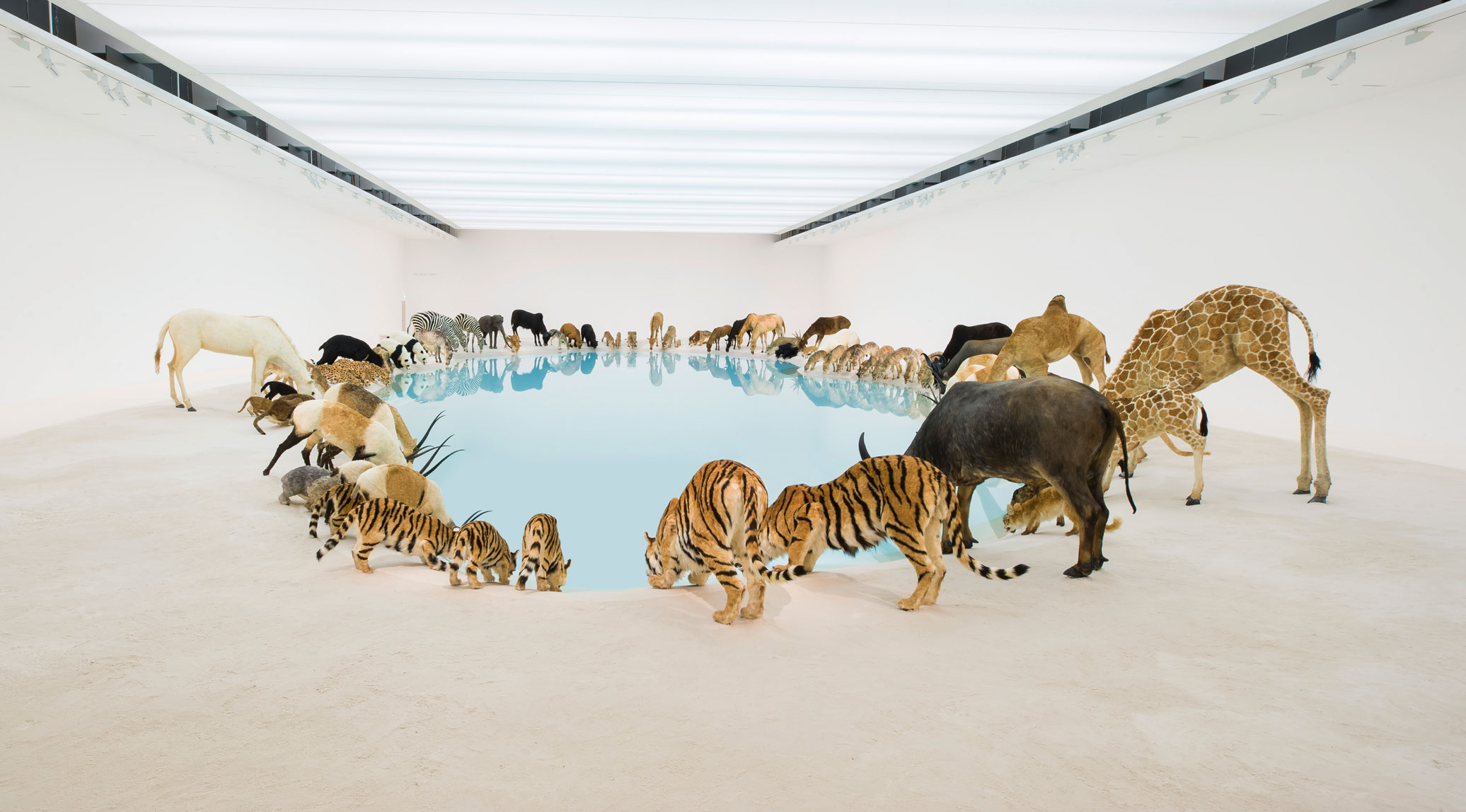The image presents a highly realistic painting depicting the interior of a spacious, artificial room with white walls and a bright, light-filled ceiling. At the center of the room is a circular pond or pool filled with blue water, around which a diverse array of animals congregate, as if drinking simultaneously. The floor surrounding the pond is a bare tan color, adding to the room's stark, minimalist appearance. Among the animals visible are lions, tigers, giraffes, horses, deer, dogs, zebras, pandas, hyenas, bulls, cows, and camels, all standing side-by-side. The scene is surreal, given the unnatural setting and the variety of species, more akin to a jungle or savanna, all captured in a single moment.